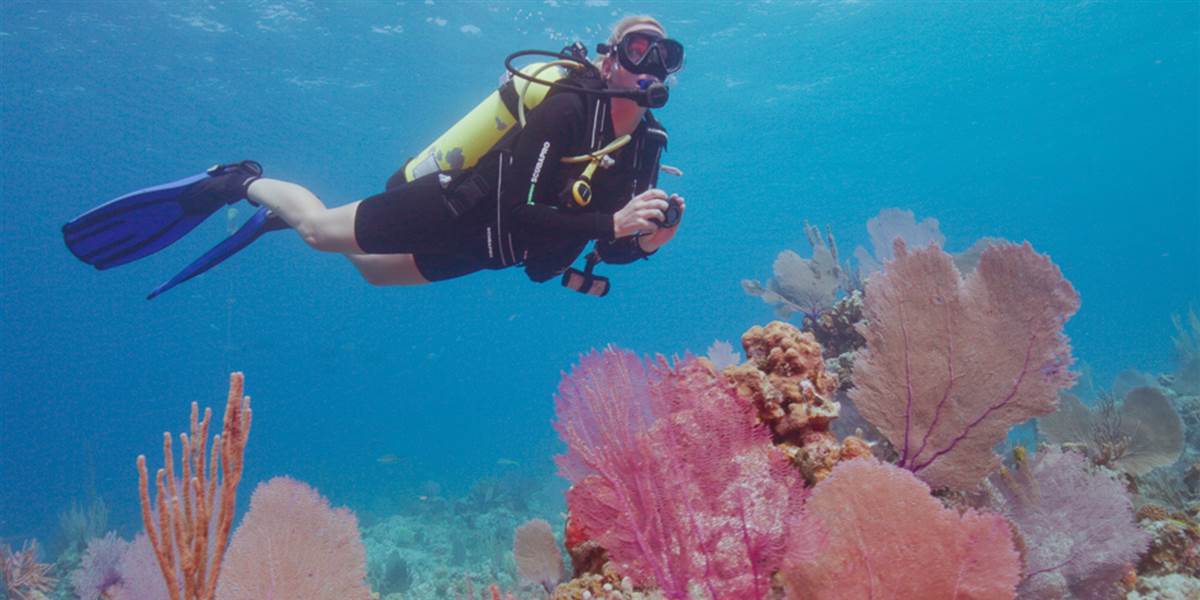The image captures an underwater scene with a scuba diver photographing a vibrant coral reef. The diver, clad in a black suit with shorts and blue flippers, is focused on the seafloor while holding a small camera with both hands. He wears red-tinted black goggles and a large, neon yellow oxygen tank connected to his mouth by a black hose. The tank is additionally emitting some air bubbles as he moves. The background is a serene blue with light rays penetrating the water, illuminating the scene. The diverse coral reef below is detailed and colorful, featuring purple fan-like plants among yellow rocks and a range of coral from peach and pink to more orange shades. The diver’s head is towards the top center of the image, facing downward towards the coral, capturing the beauty of the underwater ecosystem.